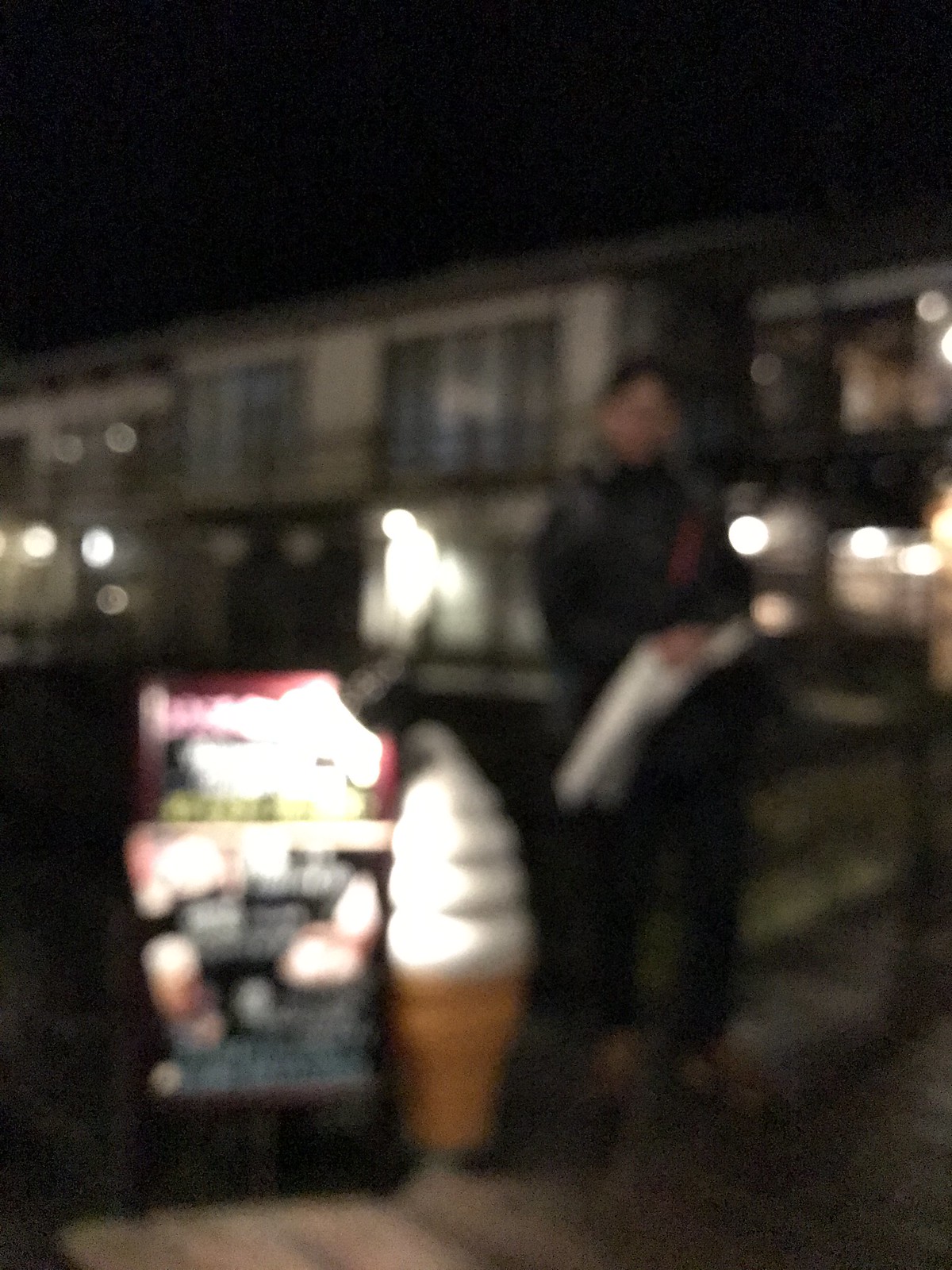In this nighttime photograph set in a residential area, the camera’s motion and shake have produced a blurred, out-of-focus image. The central focus of the picture is a brightly lit ice cream vendor cart. At the base of the cart, a large model of a swirled soft-serve ice cream cone draws immediate attention. The cart itself is adorned with illuminated signs on its sides. Beside the cart stands a man, likely the vendor. In the background, the scene is framed by two-story residential buildings, their details hazy due to the image’s lack of sharpness. The ambient light from the cart suggests it may be powered by a generator, adding a whimsical nocturnal charm as it peddles ice cream products in the stillness of the night.